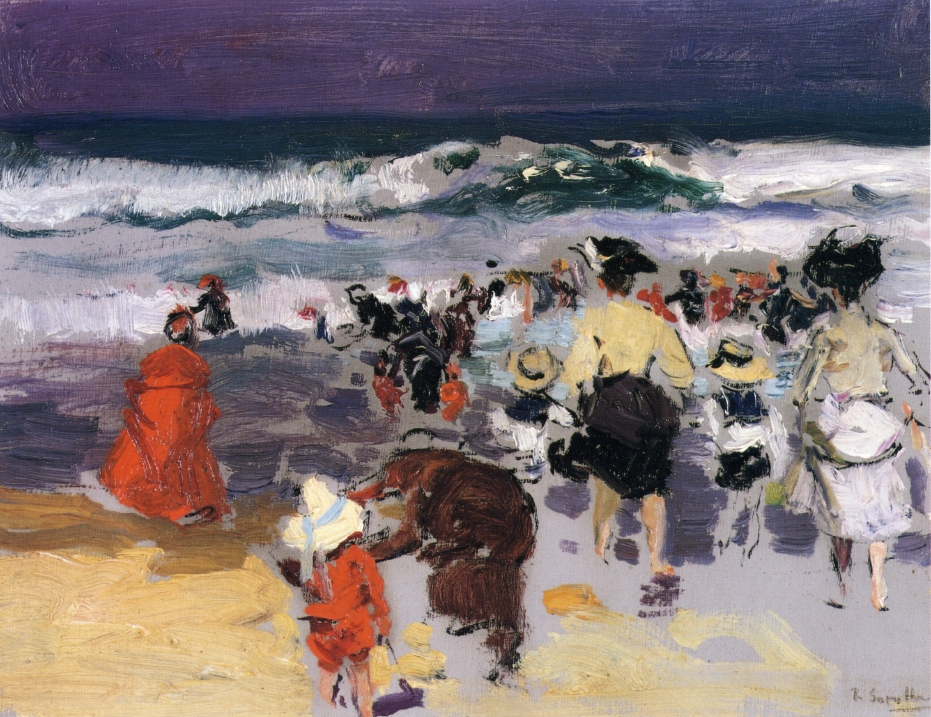This image is a highly impressionistic painting depicting a beach scene, primarily featuring women and children. The painting employs a mostly dark palette with primary colors such as black, white, red, yellow, brown, and muted tones of tan, brown, orange, purple, gray, and dark green. The center of the image prominently features a group of people walking on the sand towards the ocean waves, which are seen crashing in the background under a black starlit sky. Some women are lifting their skirts to avoid getting them wet, and they are adorned with large feathered hats. The children are dressed in black, white, or red outfits with woven hats. One notable woman wears a striking red robe. The individuals closer to the viewer are more detailed, whereas those near the waves are more abstract and impressionistic, suggesting the form of human figures without intricate details. There is no text in the image, but a signature from the artist is visible in the bottom right corner. This piece, evocative of museum or art show quality, encapsulates a vivid yet abstract portrayal of a moment at the beach.